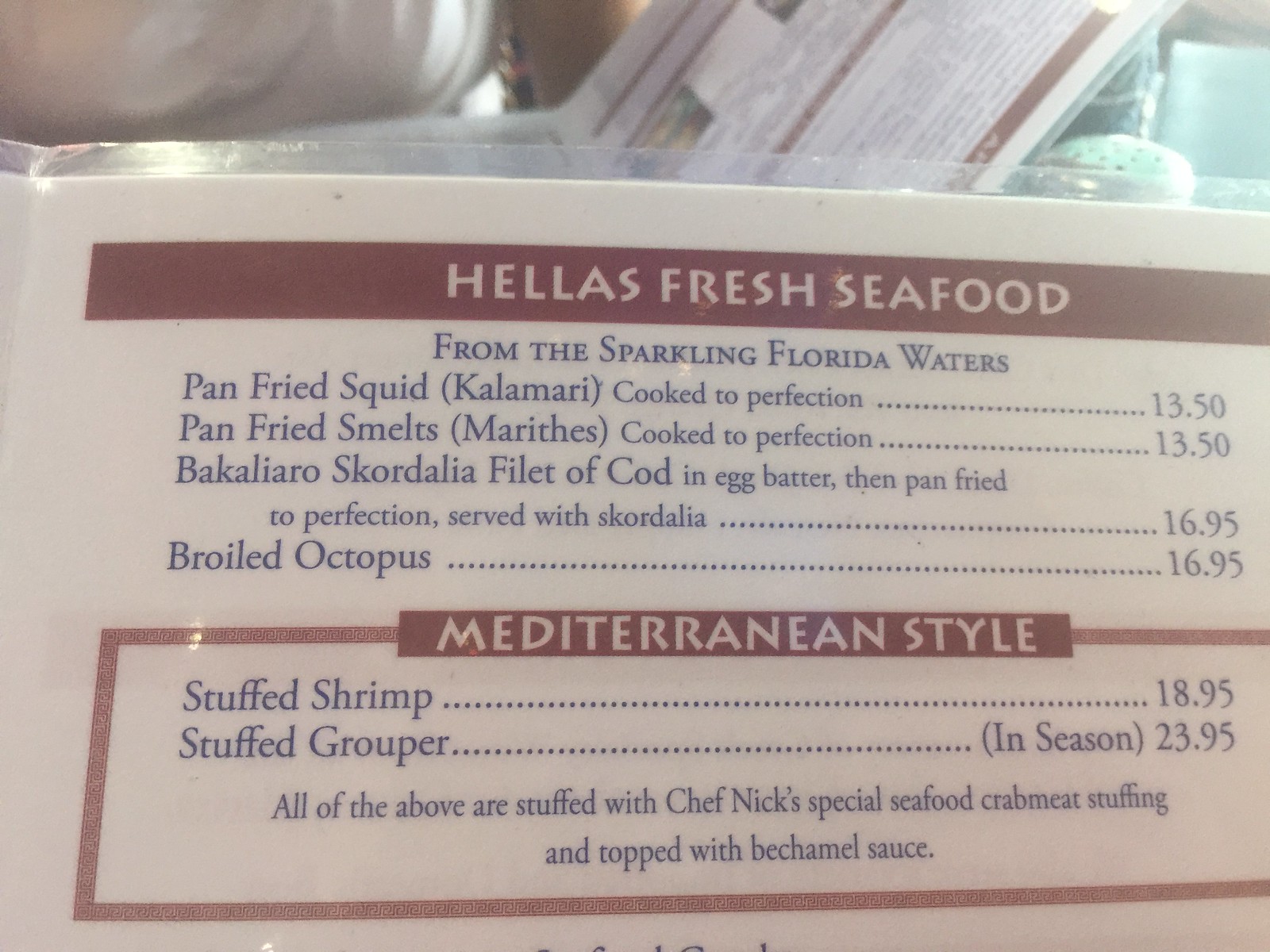This indoor image features several distinct elements. In the upper left corner, there is an unidentified object of a silvery-white hue. Moving rightward, near the center, a main feature of the image emerges—a laminated seafood menu. In the upper right area, another unidentifiable gray object sits near a rounded gray item.

The focal point of the picture is the detailed seafood menu. The laminated white paper displays visible clear laminate along the top edge. A prominent gray rectangle at the top reads "HELLA'S FRESH SEAFOOD" in bold lettering. Below, in black text, a description follows: "From the sparkling Florida waters." The menu lists several seafood dishes with prices. Firstly, "Pan Fried Squid (Calamari), cooked to perfection, $13.50." Next, "Pan Fried Smelts (Marthids), cooked to perfection, $13.50." Another dish is "Filleted Cod in Egg Batter, then pan fried to perfection, served with Squirtolini, $16.95," though the name "Squirtolini" might not be clearly identified. Lastly, "Broiled Octopus, $16.95."

Also featured is a brown square, inside of which, "Mediterranean style" is written in white text. Below this square, in black font, the menu lists "Stuffed Shrimp, $18.95" and "Stuffed Grouper, in season, $23.95." Under these listings, in smaller print, the menu mentions that "All the above are stuffed with Chef Nick's special seafood crabmeat stuffing and topped with Béarnaise sauce."

Overall, the image highlights a detailed and enticing selection of seafood offerings, carefully described and attractively presented.